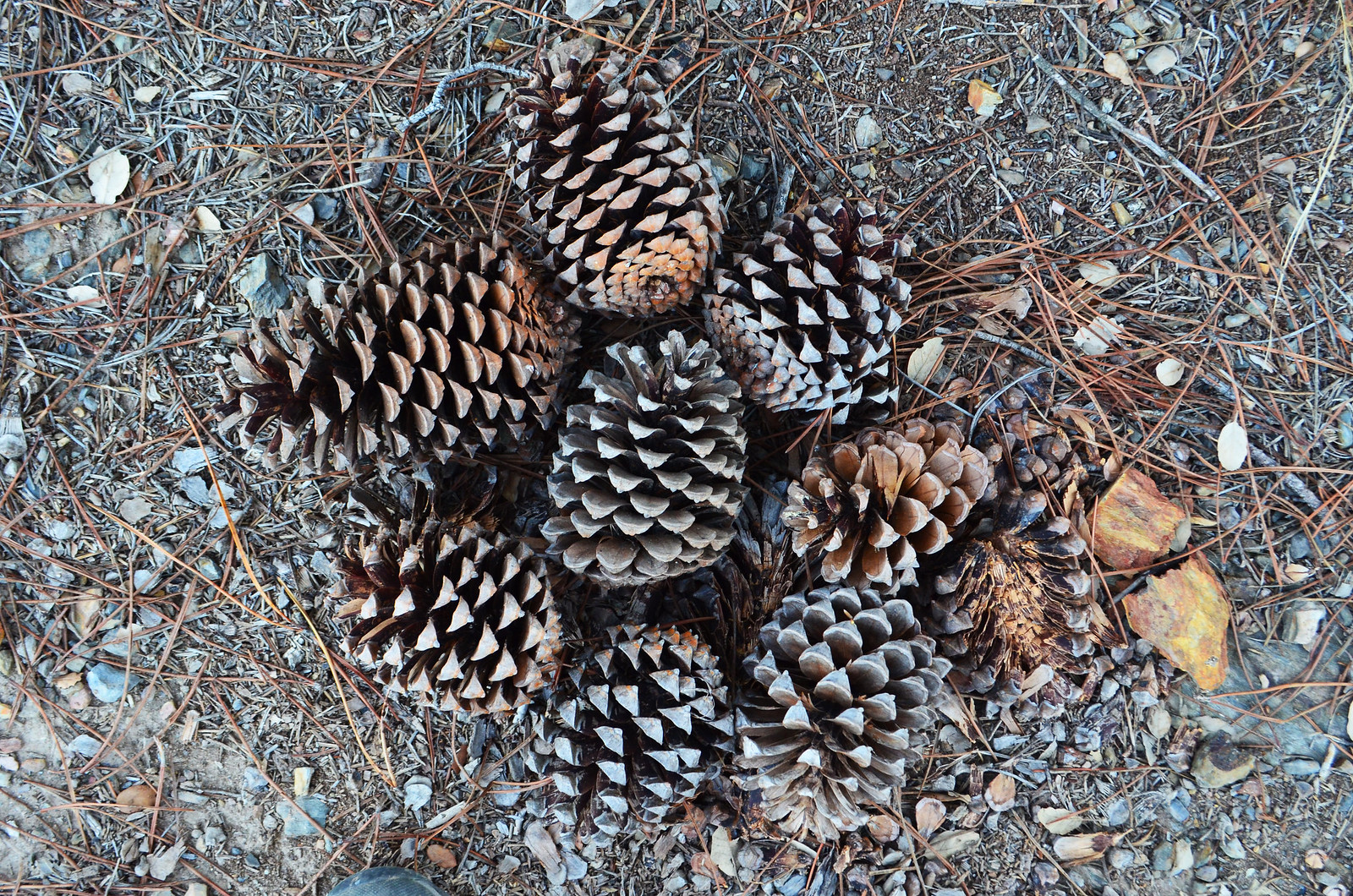This is an outdoor photo of a forest floor covered with dirt, pine needles, leaves, small stones, and broken twigs. In the very center, nine pine cones are carefully arranged in a circular pattern, with one medium-sized pine cone at the center. Surrounding it, the other eight pine cones have their bases pointing inward and tops facing outward. The pine cones vary in color from light brown to grayish white, with one notably damaged pine cone appearing almost bald on one side. At the bottom left of the image, a small portion of the photographer's left shoe is subtly visible.